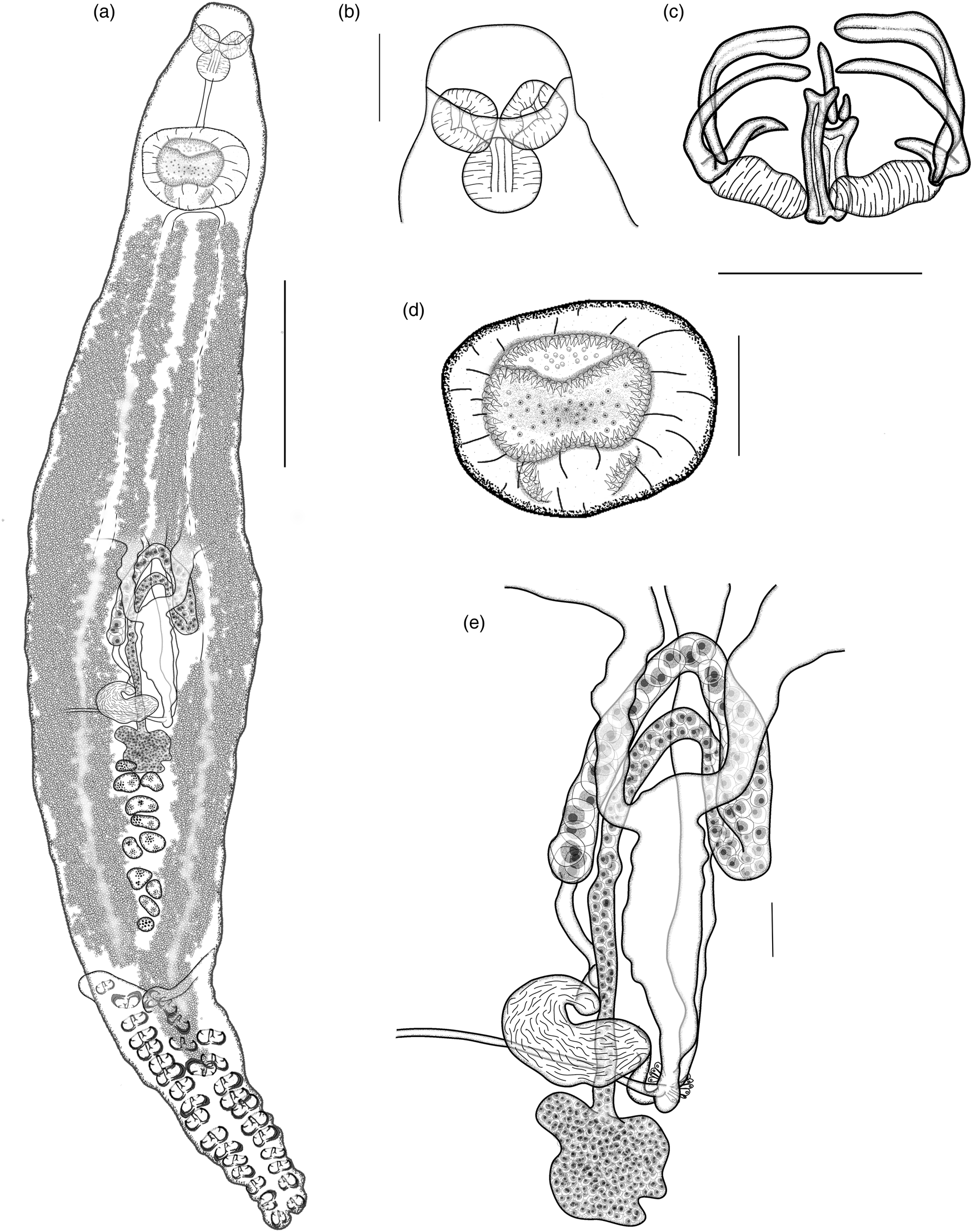The image is a hand-drawn, black-and-white diagram featuring five distinct structures labeled A, B, C, D, and E. The diagram appears to illustrate different cellular or molecular forms, starting with an overview and then zooming in to detail the individual components.

Structure A, which runs from the top to the bottom of the drawing, resembles an elongated shape similar to a banana or cucumber. It is depicted in a cross-section to reveal inner details, including a fleshy center and seed-like elements at the bottom, capped off with circular cell-like structures at the top.

Structure B, located at the center top, consists of three circles aligned with a line running over them, reminiscent of a turban shape. 

Structure C, positioned at the top right, vaguely resembles seaweed or a crab with pincers due to its intricate, branching form.

Structure D, found in the middle, features a simple, fried egg-like shape, representing another cell structure.

Structure E, situated in the lower left corner, is the most abstract, bearing an appearance likened to fallopian tubes or an alien drawing, giving an impression of complex, unidentifiable morphology.

Despite the lack of labels, the diagram presents a detailed depiction of various cell-like structures, focusing on their unique shapes and internal configurations.